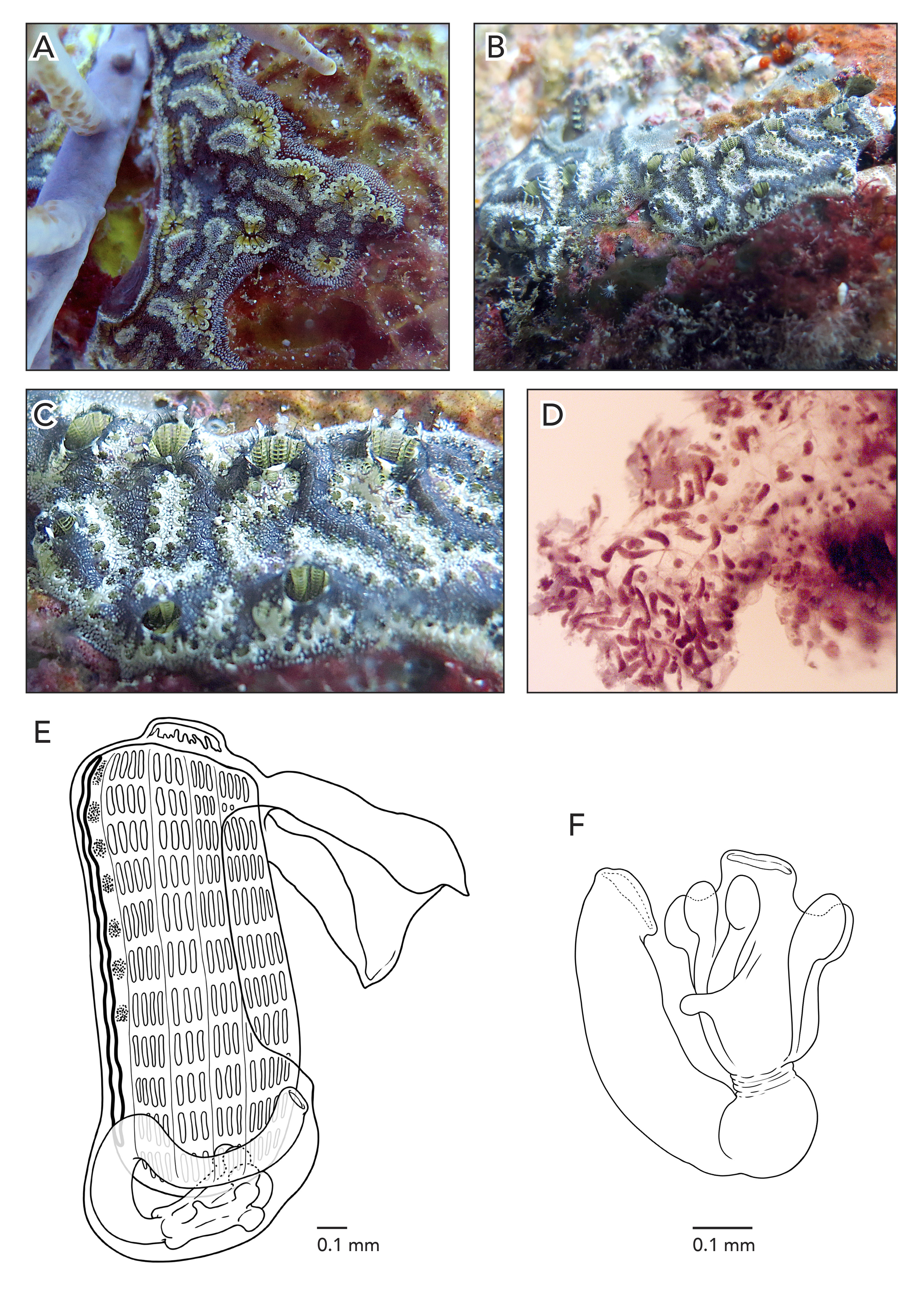The image consists of six labeled sections A through F, depicting what appears to be various forms of coral and marine life. The top four sections A, B, C, and D each showcase different coral formations. 

In section A, the image displays a bluish-gray coral adorned with green and yellow polyps scattered around its surface. Section B features a blue and white coral structure, echoed in section C but in a more zoomed-in view, revealing intricate details of the blue coral and tiny green spots. Section D stands out with its pinkish-purple hues and delicate lines against a more reddish or tan pink background.

Sections E and F differ from the coral images, presenting black and white line drawings. Section E illustrates a tube-like structure, while section F likely depicts another tubular organism or plant. Both sections are marked with a scale, indicating a size of 0.1 millimeters, suggesting these are detailed scientific diagrams, potentially from a biology textbook.